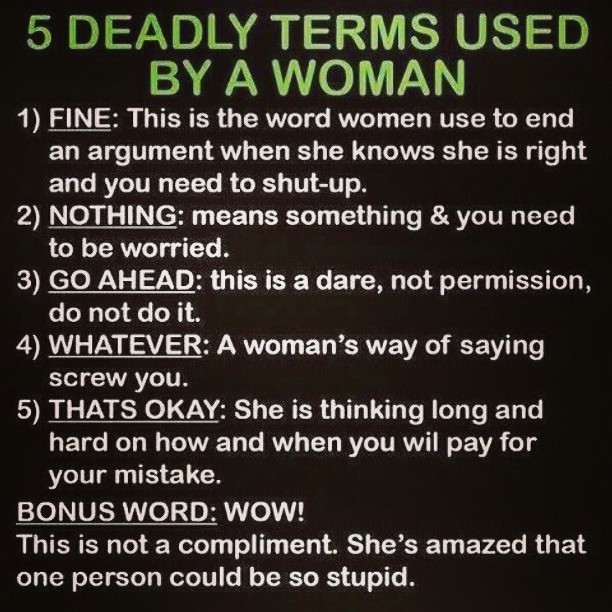The image features a black background with bold text providing a humorous guide on "5 Deadly Terms Used by a Woman." At the top, the title is displayed in eye-catching lime green text. The rest of the content is in white font. The list includes:

1. **FINE**: This is the word women use to end an argument when she knows she's right, and you need to shut up.
2. **NOTHING**: Means something, and you need to be worried.
3. **GO AHEAD**: This is a dare, not permission. Do not do it.
4. **WHATEVER**: A woman's way of saying "screw you."
5. **THAT'S OKAY**: She is thinking long and hard about how and when you will pay for your mistake.

At the bottom, a "BONUS WORD" is highlighted:
- **WOW**: This is not a compliment. She's amazed that one person could be so stupid.

Each term and the bonus word are bolded and underlined, making the guide easy to follow. The overall presentation suggests that the image is a digitally created piece, possibly shared as an instructional or humorous post to help understand nuances in women's speech.